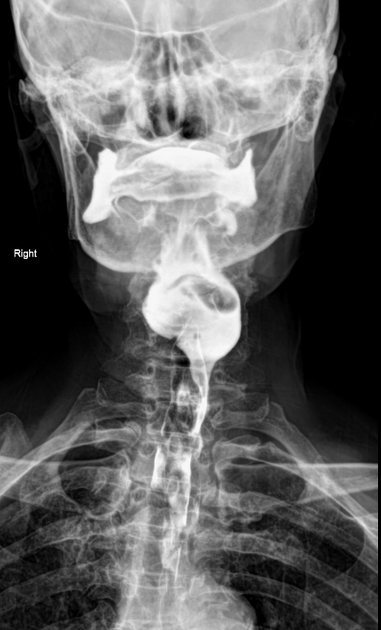This detailed black and white x-ray image captures the top portion of a person's body, from roughly two-thirds of their head down to just below their chest area. The skeletal structure, including the skull, neck, shoulder bones, and parts of the ribcage, is outlined in shades of gray and white against a stark black background. Despite some ambiguity among observers, it seems likely that the image is captured from the back of the person, given the prominence of the skull and the absence of visible eye sockets.

A peculiar and striking feature within the neck stands out prominently: it appears as a large, circular object, resembling a "tube of sushi" in some descriptions, that seems out of place in the anatomical structure. Additionally, another observer noted what seems like a rectangular plate with small handles near this area.

The only text in the image is the word "right," situated on the left-hand side of the x-ray, adding an element of confusion. This might indicate the image's orientation but remains unclear due to positioning. No additional people or elements are present in the x-ray, ensuring the focus remains on the intriguing and perhaps concerning features within the neck and the rest of the upper body anatomy.